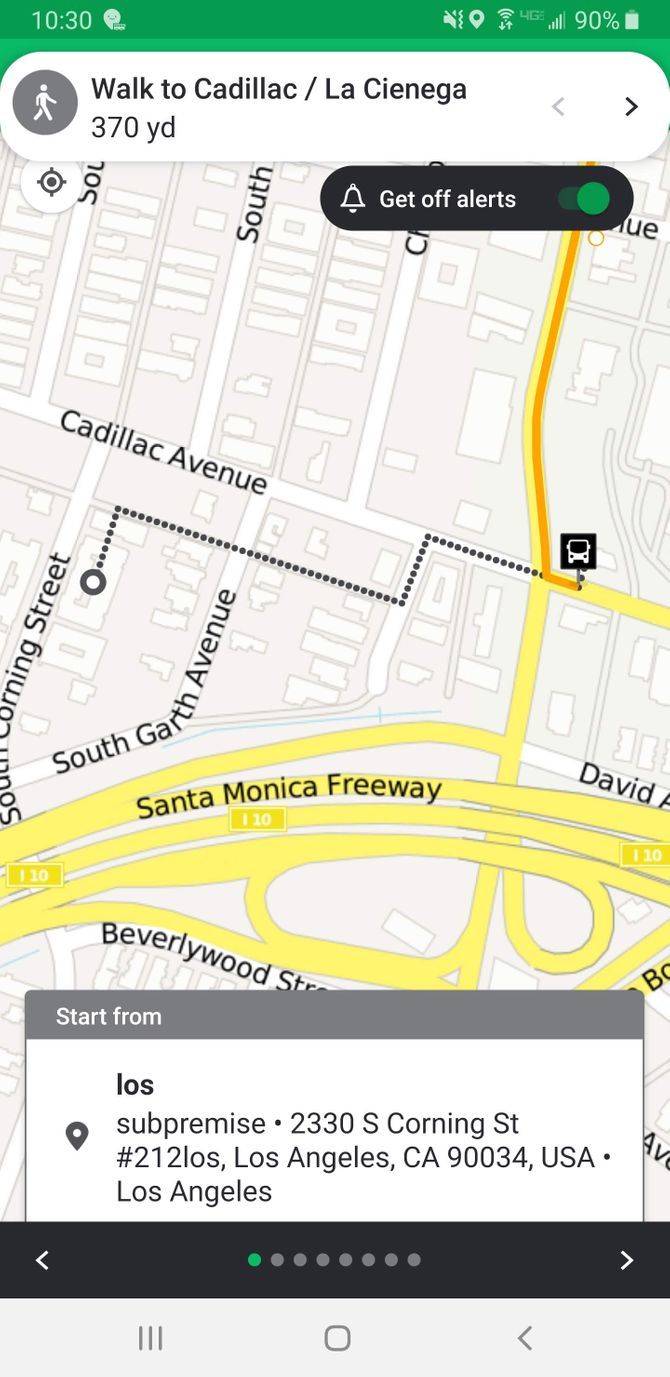A detailed screenshot captured from a mobile device shows a user navigating with a maps application, most likely Google Maps. The interface prominently displays a partial map where a highlighted route is visible, suggesting the planned path the user intends to take. This is unmistakably a mobile screenshot, as evidenced by the top left corner of the screen showing the time, 10:30, along with icons indicating strong cell signal, Wi-Fi connectivity, and a battery level at 90%.

The map features a background in shades of gray, with roads and buildings outlined, along with street names clearly labeled. The route is marked in multiple colors—yellow, green, and orange—indicating various traffic conditions along the path. The user is starting their journey from 2330 South Corning Street in Los Angeles, California, 90034, USA. Their destination is 370 yards away, suggesting a brief walk to a location near Cadillac Avenue or La Cienega Boulevard. The path suggests the user will be moving towards Cadillac Avenue, providing a concise guide for the short journey within the Los Angeles area.